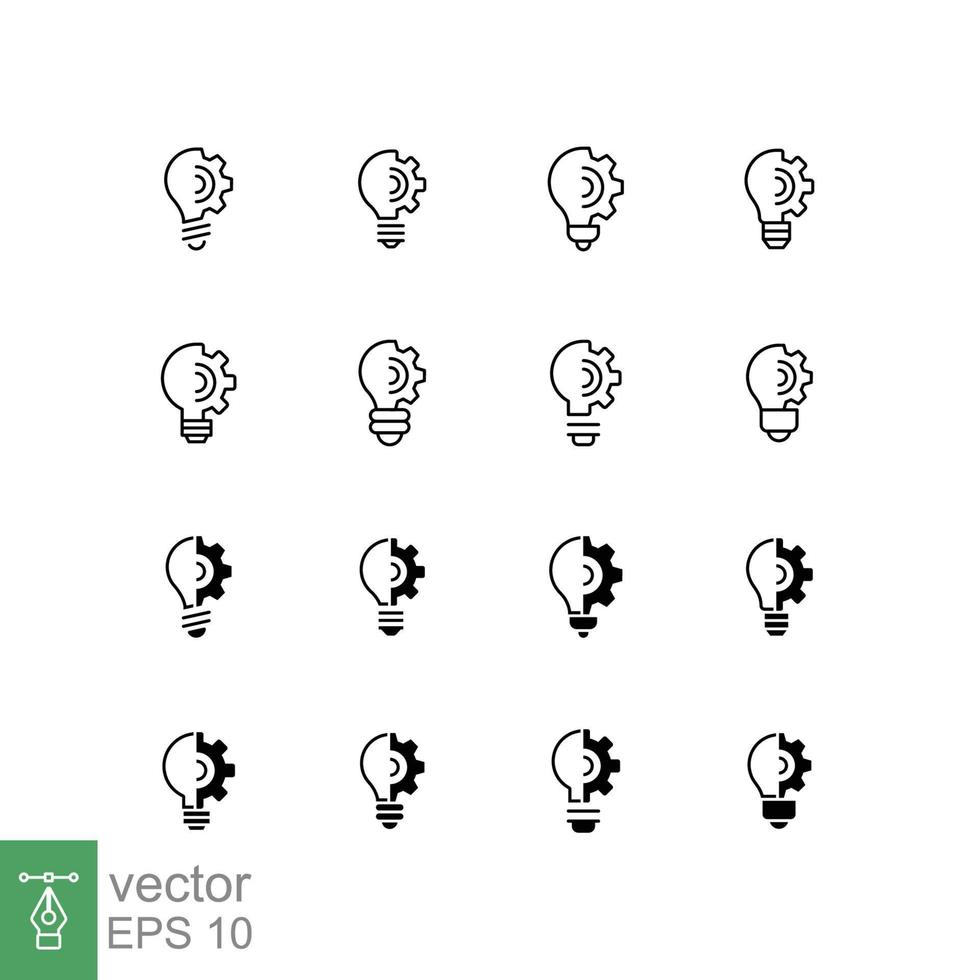The image features 16 vector illustrations, organized in four rows of four. Each illustration represents a half light bulb, combined with a mechanical gear or screw icon. The top two rows present the images in line art, while the bottom two rows depict the right side of each light bulb and gear icon filled in solid black, with the screw-in portion also varying in shading from light to dark as you move downward. In the bottom left corner, there is a green rectangle containing a white symbol that resembles a pinhead with three points aligned above it. Next to this symbol, the text "Vector EPS-10" is displayed in gray font.